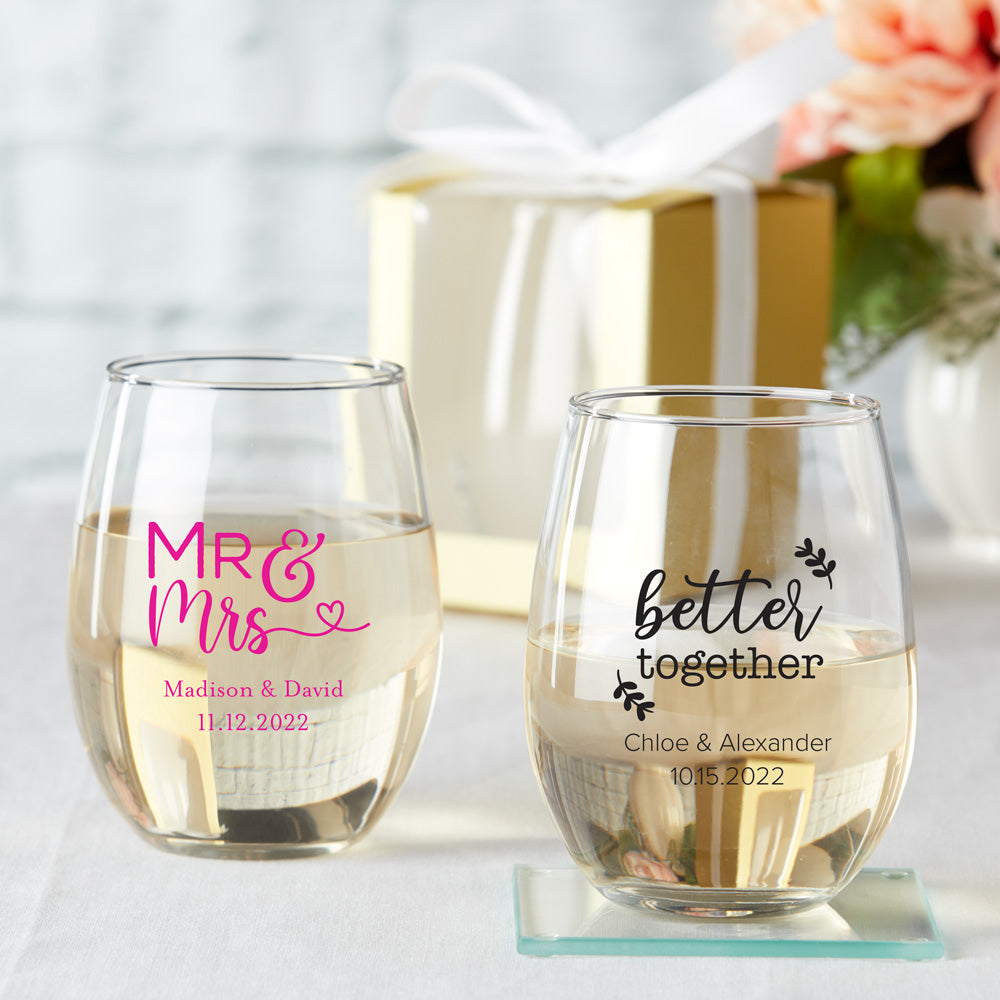In the large, square image with no border, two stemless wine glasses are prominently featured on a white surface. The glass on the left, slightly behind the one on the right, is inscribed in dark pink with the words "Mr. and Mrs." followed by "Madison and David" and the date "11.12.2022." The glass on the right, positioned slightly in front and sitting on a small transparent glass plate, bears the words "Better Together" in black, decorated with two leafy designs. Beneath the phrase, it reads "Chloe and Alexander" and the date "10.15.2022." Both glasses are filled halfway with a light tan liquid, likely champagne. In the background, there is a blurred gold, cube-shaped package adorned with a white ribbon, and a white vase containing pretty coral-colored flowers and green leaves visible in the upper right corner.